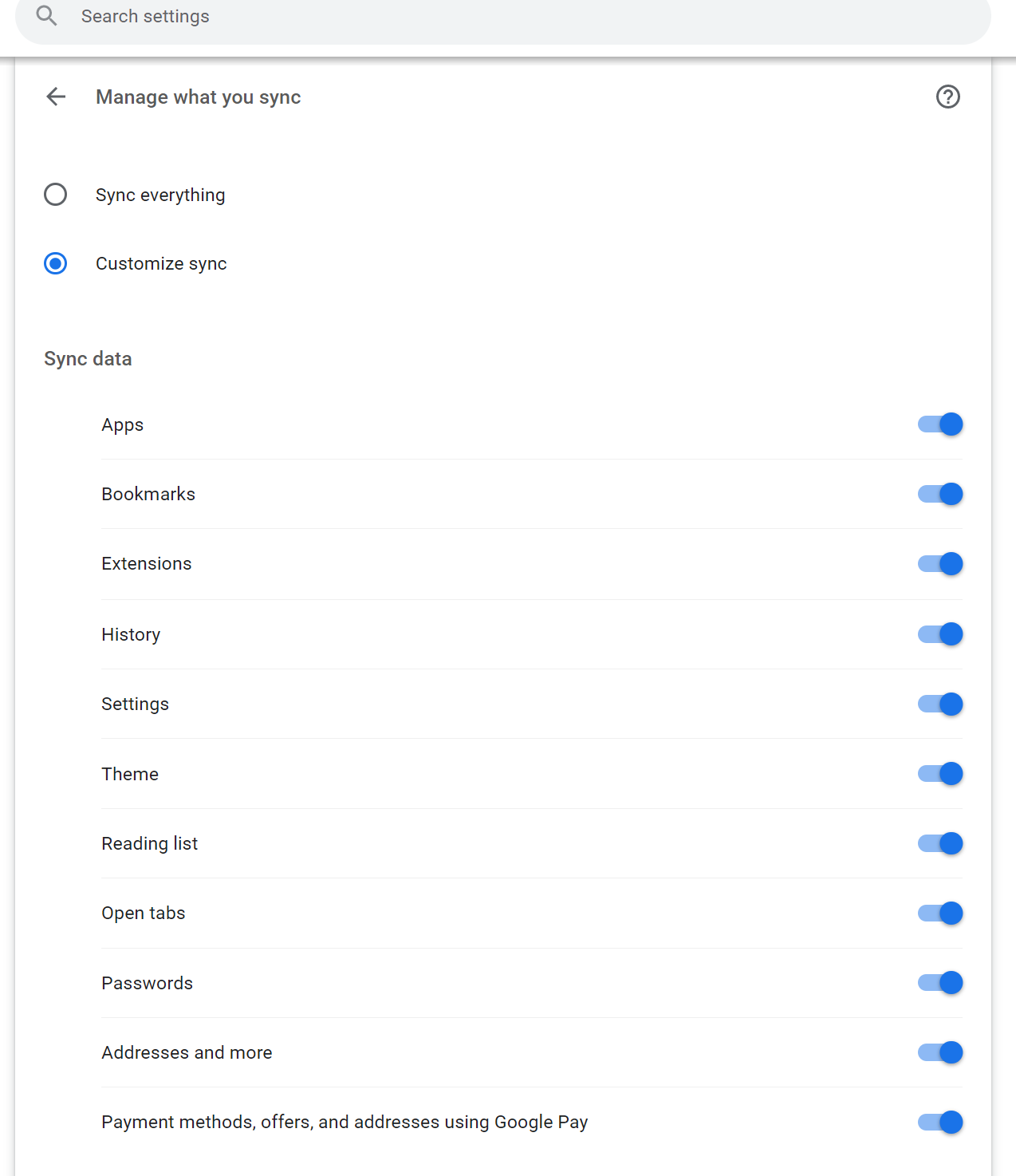This rectangular image is vertically oriented, with its longer side extending from top to bottom. At the very top of the image, a gray, oblong search box is situated, featuring a search icon on the left side and the text "Search settings" next to it. Below this search box is a thin gray line acting as a separator.

Parallel thin gray borders run down both the left and right edges of the image. Directly beneath the separator is a black arrow pointing to the left labeled "Manage what you sync." On the far right of this same row is a white circle with a black outline enclosing a question mark.

Below the "Manage what you sync" row are two radio buttons. The first radio button, a white circle with a black outline, is labeled "Sync everything." The second option, indicated by a blue circle with a blue outline, is labeled "Customize sync."

Further down, the text "Sync data" introduces a list of items, each marked with a radio button on its right side and separated by thin gray lines. The list includes:

- Apps
- Bookmarks
- Extensions
- History
- Settings
- Theme
- Reading list
- Open tabs
- Passwords
- Addresses and more

At the bottom, additional items are mentioned: "Payment methods, offers, and addressing using Google Pay."